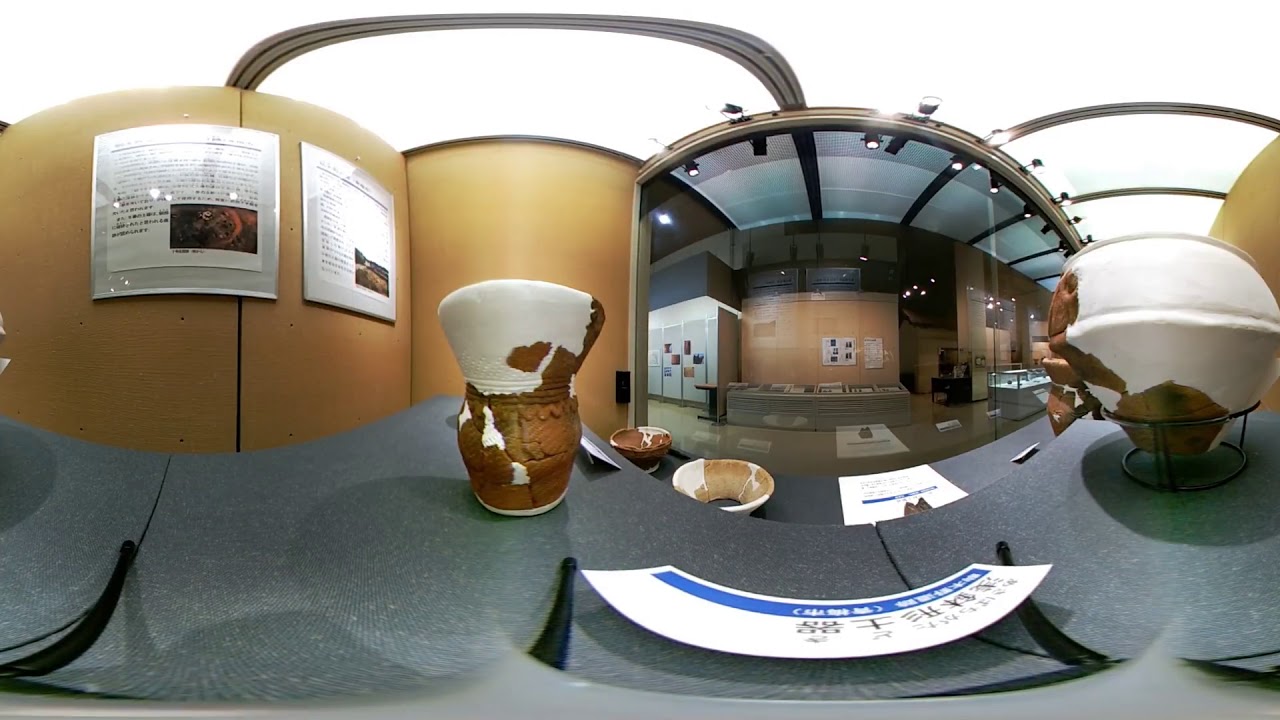Captured through a fisheye lens, this image appears to be set within a sophisticated lobby, likely belonging to a history museum or a similar establishment. Dominating the left side of the frame is an intricate ceramic vase. The vase, primarily brown, bulges prominently at the bottom and is adorned with detailed designs. Its upper portion is largely covered in white paint, and it rests on a gray table. In front of the table lie two ceramic bowls: the left one dark brown and the right one a lighter shade, both featuring white paint accents.

Adjacent to the vase on the gray surface is a white piece of paper with a blue strip at the top and black text in a foreign language, likely Chinese. To the far right, another display features what looks like a globe or a decorative ball supported by a black stand, with brown and white paint dominating its surface, and a touch of green at the base where it meets the stand.

Further back, you can see through a pane of glass into another room with a brown wall, a gray desk, and banners hanging on the wall, which are white squares with writing, possibly informative. To the left of this desk is a white wall adorned with hanging pages. The fisheye lens distorts the far-left side of the image, making the light brown wall appear rounded, featuring two square displays with a shiny finish and documents including pictures and text written in a foreign language.

The ceiling above is bright white, illuminated as if light is shining through. Silver arches stretch across the ceiling, with one on the left side and two on the right, adding a touch of modernity to the scene. Overall, this visually rich setting combines elements of pottery, textual displays, and historical artifacts, all suggesting an environment devoted to cultural or historical exhibitions.